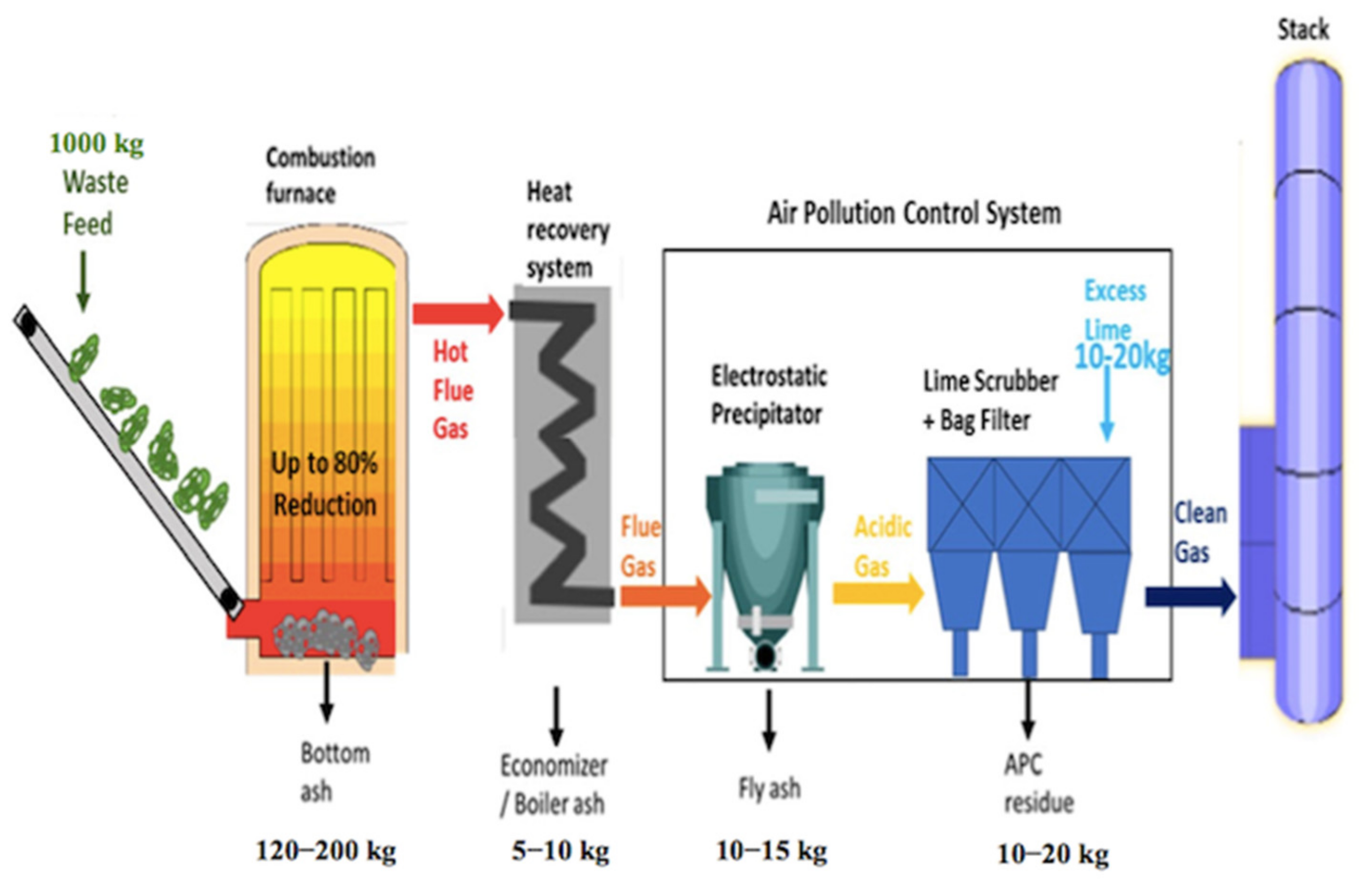The image is a detailed, brightly-colored diagram of an air pollution control system, illustrated in a cartoon-like or computerized style. It maps out the journey of 1,000 kilograms of waste feed through several key stages. The waste feed enters a combustion furnace, achieving up to an 80% reduction in volume, resulting in ash at the bottom. Hot flue gas produced during combustion goes into a heat recovery system before proceeding to an air pollution control section. Here, it passes through an electrostatic precipitator, generating fly ash, and then through a lime scrubber and bag filter, producing APC residue and excess lime. Finally, clean gas is released through a purple smoke stack. Each component, from the initial waste feed to the final clean gas emission, is meticulously labeled, with corresponding kilogram reductions noted at various stages: from 1,000 kg to intermediate weights of 120-200 kg, followed by 5-10 kg, 10-15 kg, and 10-20 kg. The diagram is visually engaging with vivid colors, including blues, greens, grays, blacks, oranges, and yellows, and is likely intended for educational purposes, possibly as part of a book or a poster.